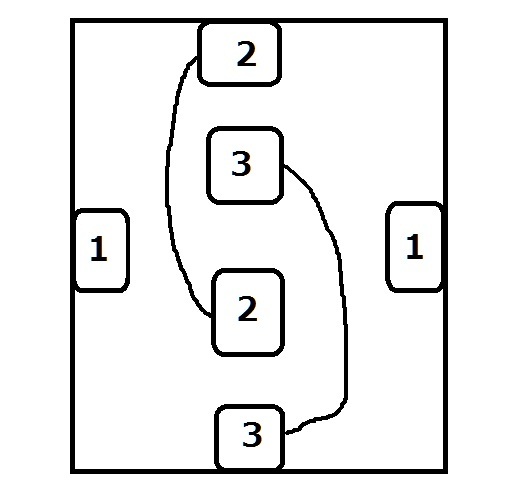A meticulously crafted black-and-white graphic image, created digitally, featuring a larger square frame containing six smaller, numerically labeled squares. Starting from the top, each square is sequentially positioned as follows: At the top center is square 2, directly below it sits square 3. Beneath square 3 is another square labeled 2. At the very bottom center of the image lies the final square labeled 3. Additionally, two squares labeled 1 are placed towards the edges: one on the center-left and another on the center-right side of the image. A bold line connects the top square 2 with the middle square 2 on the left side, while another line links the second square 3 with the bottom square 3 on the right side. The entire composition utilizes a stark black and white color scheme, emphasizing the structural and numerical relationships between the squares.